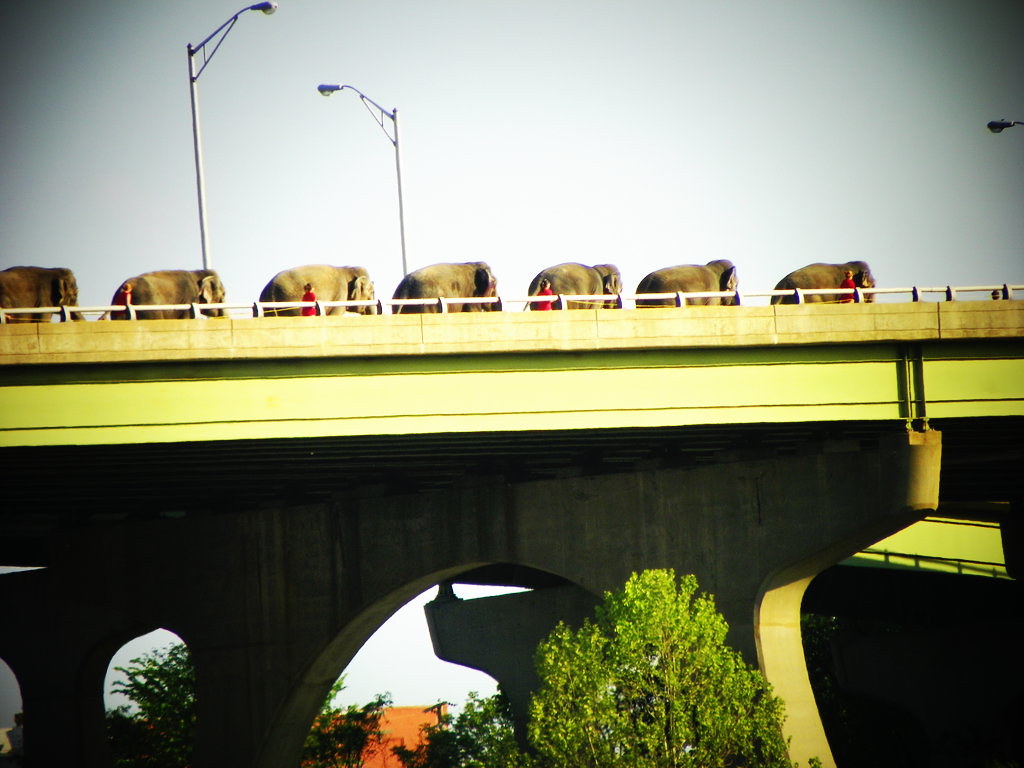In this bright outdoor photograph, a large gray concrete bridge with a distinctive arched support underneath spans the entire width of the image. The bridge features white rails held up by small white posts along its sides and is adorned with three gray street lamps—two positioned towards the middle and one on the far right. Walking in a straight line across the bridge from left to right are seven large gray elephants, distinguished by their big floppy ears, long trunks, and humped heads. They are accompanied by four people: three in red shirts and one in a black shirt or tank top. Below the bridge, lush green trees are visible along with the orange roof of a distant red building. The sky above the scene is bright, almost white, adding to the vividness of the day.